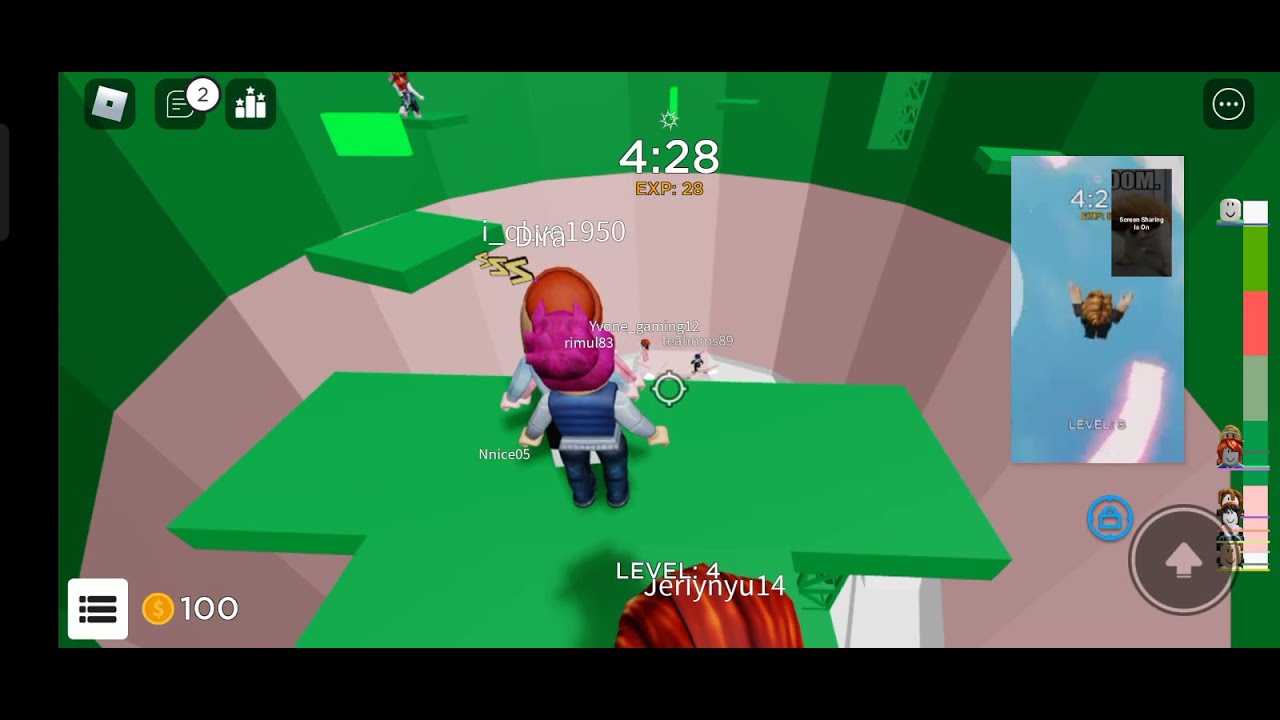In this full-color screenshot from the video game, we see a vividly detailed cylindrical room with a uniquely colorful design. The room features lower panels in shades of pink and upper green sections, bordered by a thick black edge on three sides. At the center, two players, distinguishable by their orange and pink hair respectively, are positioned on a floating green platform made up of two rectangles, possibly standing on the head of a third, obscured player who has a brown cap. The players, dressed in blue vests over white-blue long-sleeved shirts and blue pants, are engaged in gameplay that involves jumping around this dynamic world. Above the players are their in-game names in white text.

The screenshot also displays various HUD elements. The top center shows a countdown timer reading 4 minutes and 28 seconds, accompanied by an "EXP" score of 29. A level 4 indicator is also visible. There's an inset map of another game area, a vertical progression bar on the right with a strip scaled in colors from pink to green and several icons surrounding the main display— including a coin symbol indicating 100 coins and a message icon with the number 2. This descriptive image captures an immersive blend of gameplay mechanics and colorful visuals.